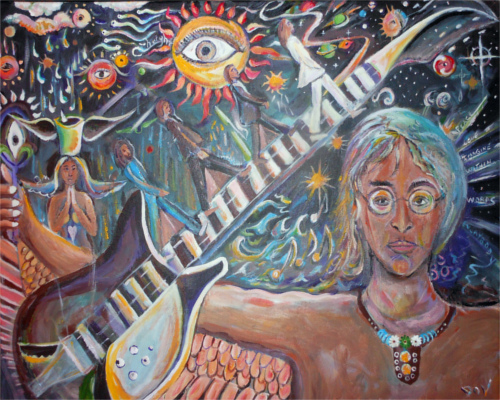The image is a striking modern painting featuring a multitude of elements and vibrant colors. At the bottom right corner, the figure of a man strongly resembling John Lennon stands out, characterized by his iconic round glasses, long skinny face, and necklace adorned with a large brown pendant, blue beads, and white daisies. John's arms are outstretched, and he is shirtless, possibly holding a plant in his right hand. Nearby, an electric guitar is positioned with its body in the bottom left corner, tilting diagonally upwards to the right, crossing over John's head. The neck of the guitar is detailed with white frets and dark colors, accented with yellow and green hues.

Walking along the neck of the guitar in a fashion reminiscent of the famous Abbey Road photo, four figures that look like the Beatles march in uniform. Above them, in the top center of the painting, an orange sun with a white eye gazes out, surrounded by red rays. The background is a lively mix of colors and shapes, including circles, rainbow hues, stars, planets with rings like Saturn, and feathered wings near John's right arm. Additional details such as a cup with droplets or tears and swirling waves further enrich the scene, creating a complex, multifaceted artwork that captivates with its depth and symbolism.